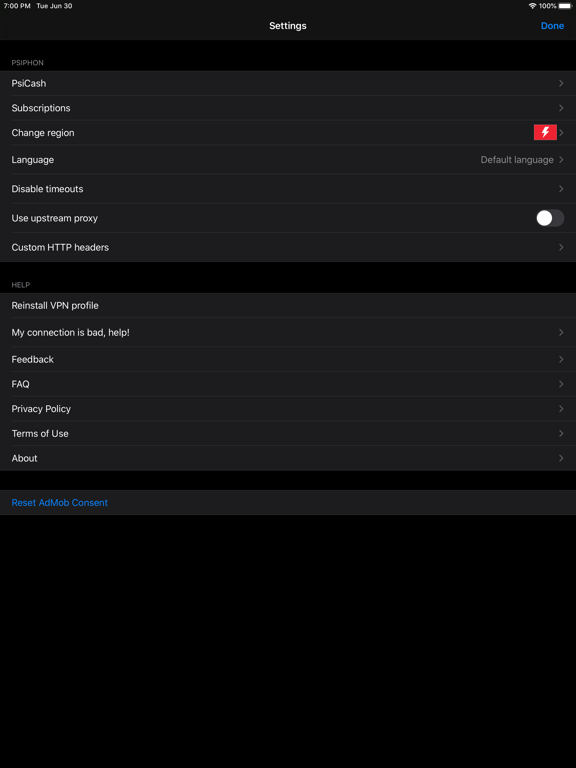This screenshot displays the settings page of a mobile application, likely running on an Android device given the layout and UI elements. The interface is set in dark mode, featuring a sleek black and dark gray background.

The settings page offers a variety of options organized under different sections:

1. **Primary Settings:**
   - **PSI, PHON, Syphon:** These seem to be features or modules managed by the app. 
   - **Sycache:** Possibly related to caching settings.
   - **Subscriptions:** Manage or view current app subscriptions.
   - **Change Region:** Option to switch regional settings.
   - **Language:** Modify the language preferences of the app.
   - **Disable Timeouts:** A toggle to prevent the app or device from timing out.
   - **Use Upstream Proxy:** Includes a toggle button to enable or disable the use of an upstream proxy.
   - **Custom HTTP Headers:** Allows customization of HTTP headers for network requests.

2. **Support and Information:**
   - **Help**: Provides further assistance, possibly including these options:
     - *Reinstall VPN Profile:* Option to reinstall the VPN profile.
     - *My Connection is Bad, Help:* Troubleshooting assistance for connection issues.
     - *Feedback:* Submit feedback or issues.
     - *FAQ:* Access frequently asked questions.
     - *Privacy Policy:* View the terms regarding user privacy.
     - *Terms of Use:* Information on the terms and conditions of using the app.
     - *About:* Details about the app and its version.

3. **Additional Options:**
   - **Reset Ad Mob Consent:** Option to reset advertising preferences and consent related to AdMob.

An "Exit" option labeled "Done" allows the user to save their settings and exit this page. At the top of the screenshot, a default time display is visible, a common feature on smartphone interfaces.